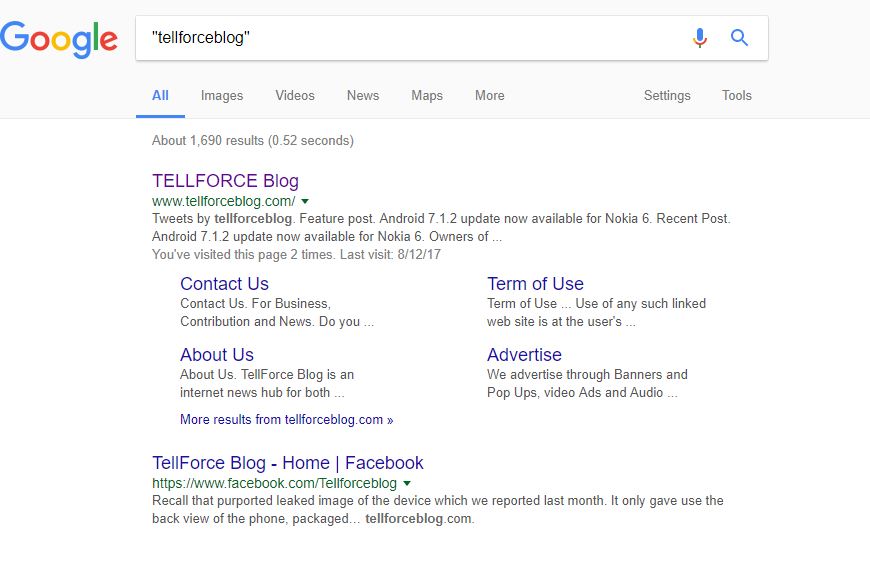The image shows a Google search results page with the query "tell false block" enclosed in quotation marks, typed in black text within the search bar. Below the search bar, the tabs for "All," "Images," "Videos," "News," "Maps," "More," "Settings," and "Tools" are displayed, with the "All" tab selected. The search yields approximately 1,690 results in 0.52 seconds.

The first result is from the website "Tell False Block," with the URL www.tellfalseblock.com shown in purple, indicating it has been visited before. The site description includes a tweet by "Tell False Block" about an update: "Android 7.1.2 update now available for Nokia 6." Notably, the page has been visited twice, with the last visit recorded on December 17.

Additional site navigation options such as "Contact Us," "Terms of Use," "About Us," and "Advertise" are also visible as blue buttons. Below the "About Us" section, there are further results linking to "Tell False Block" content, which are highlighted in blue. A related link to the "Tell False Block" Facebook page is included, with the URL displayed in green as facebook.com/tellfalseblock.